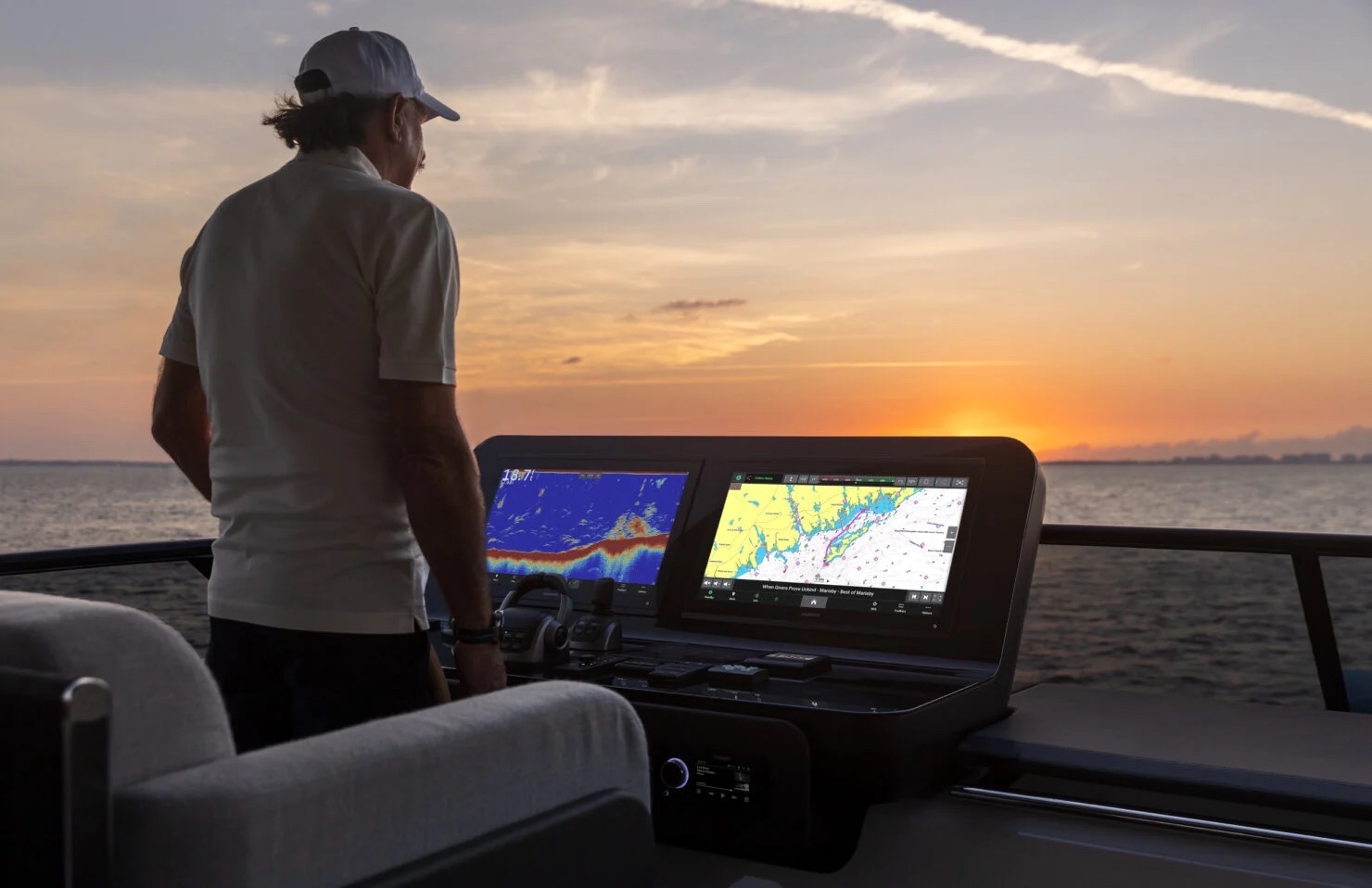In this image captured at sunset on a luxurious yacht, a man stands on the left side of the frame, facing towards the horizon on his right. He wears a white cap, a light-colored short-sleeved shirt, and dark pants, with a wristwatch on his right wrist. His left arm is bent slightly in front of him while his right arm rests at his side. He stands beside a large control panel, which features an intricate array of switches, gears, and twin display screens. One screen on the left shows a blue map indicating water depth, and the other on the right displays aerial mapping with yellow, blue, and white sections. Below the screens, various buttons and a radio dial are visible. Behind the man is a white chair with short armrests, situated on the boat's deck. The control area is sheltered by a short windshield with a black rail running across the top. Beyond the boat, the open water stretches towards the horizon with land faintly visible in the distance on the right. The sky is painted with breathtaking hues of orange, yellow, and hints of purple as the sun sets amidst scattered white clouds.